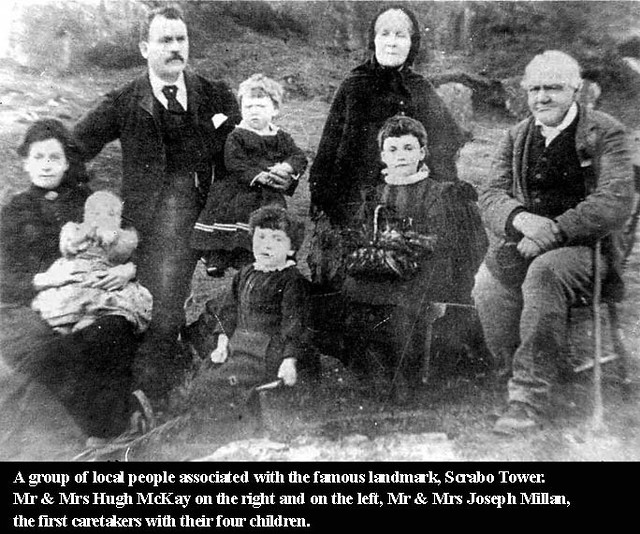The black-and-white photograph captures a group of local people associated with the famous landmark Scrabble Tower. The image is framed with a black border at the bottom, where white text reads: "A group of local people associated with the famous landmark Scrabble Tower. Mr. and Mrs. Hugh McKay on the right, and on the left, Mr. and Mrs. Joseph Millon, the first caretakers with their four children."

The photo features four adults and four children, all dressed in old-fashioned clothing. On the left, a woman sits in a chair wearing a black, high-collared dress, with a young child in a white dress perched on her lap. To her right stands a man leaning on the back of the chair, dressed in black pants, a black coat, a black vest, a white button-up shirt with a folded collar, and a black tie, with a mustache gracing his face. To his right, another woman mirrors the first, sitting in a chair with a small child on her lap. Beside these adults, two older children are seated—either on individual chairs or on the ground, dressed similarly in dark attire. The overall image has a grainy and somewhat blurry quality, yet remains clear enough to distinguish the individuals within.